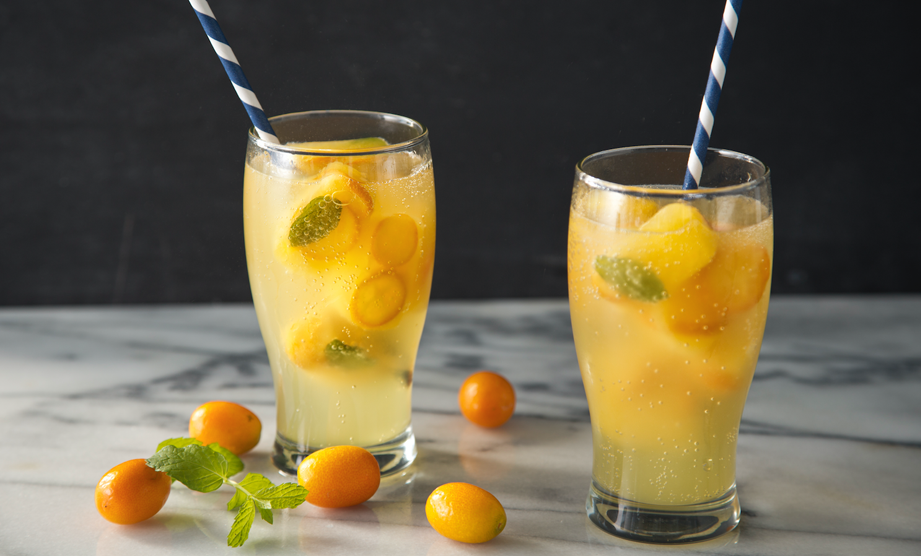This image captures two tall, clear glasses filled nearly to the brim with a vibrant, fruity beverage that resembles a blend of lemonade and orangeade. The drinks, which are perched on a marble countertop with distinctive gray swirls, are adorned with bits of citrus fruits—potentially tiny oranges like kumquats—and sprigs of fresh mint, giving them a freshly made, natural appearance. Each glass features a blue and white striped straw, adding a cheerful touch, and both contain visible bubbles, suggesting carbonation. Scattered on the countertop are additional small fruits and mint sprigs, with some of the fruits still attached to their leaves. The clear, textured glasses are subtly narrower at the base, flaring slightly towards the top, encapsulating this vibrant and refreshing scene.